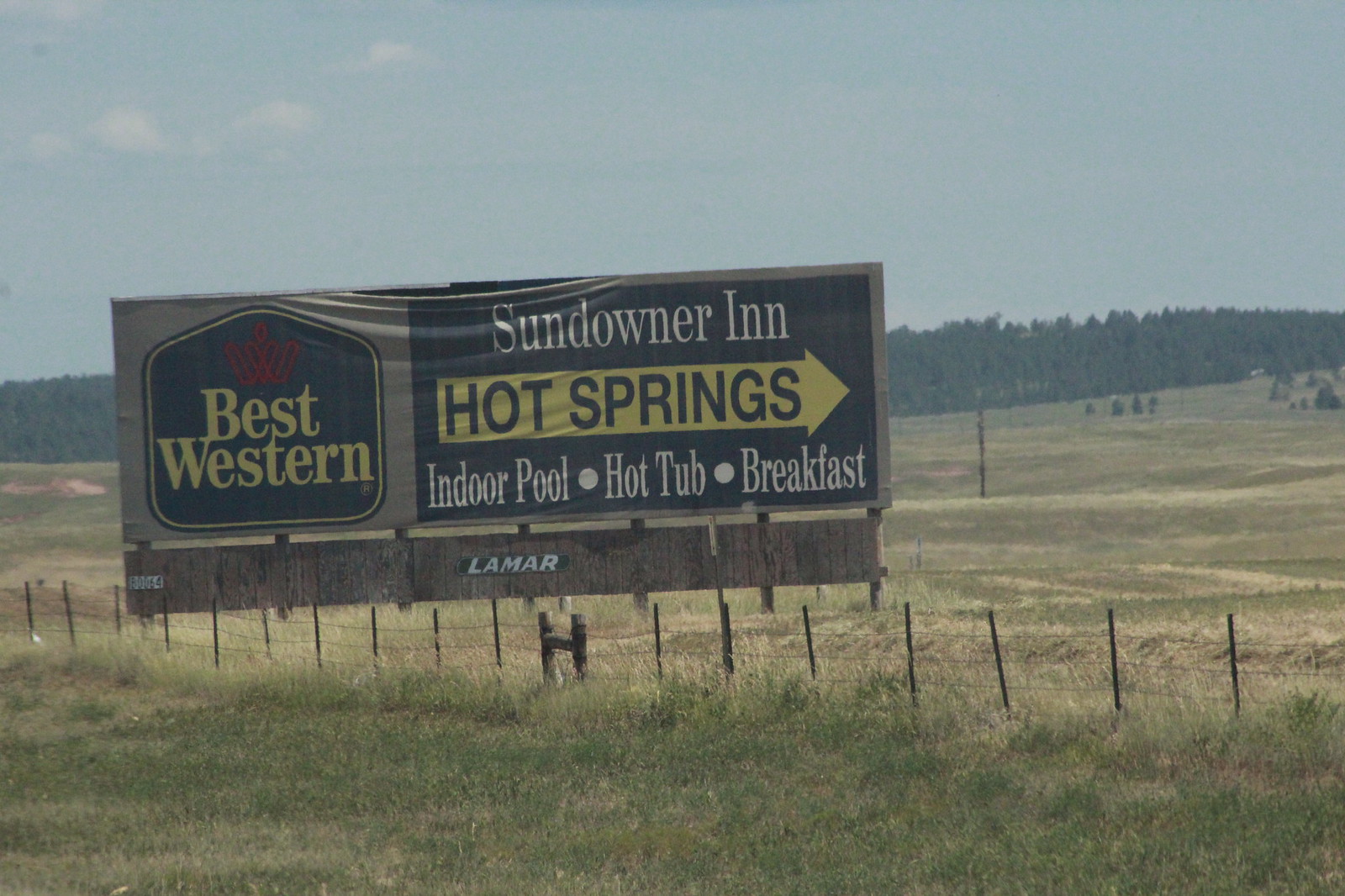This photograph captures a large outdoor billboard situated in a picturesque countryside setting, likely taken along a highway from a moving vehicle. The scene is framed by a dull blue sky with a few scattered clouds in the upper left corner. A ridgeline of trees forms the backdrop, contrasting gently with the grassy field that dominates the foreground. The field, a mix of green and yellow hues, adds a touch of rustic charm to the landscape.

The billboard is positioned toward the left side of the image, centrally placed for maximum visibility. Prominently featured on the left side of the billboard is the iconic Best Western logo. On the right side, the text reads: "Sundowner Inn. Hot Springs," with "Hot Springs" displayed in a sizeable arrow pointing to the right. Below this, additional amenities are listed, including "indoor pool," "hot tub," and "breakfast," enticing travelers to stop and enjoy a comfortable stay.